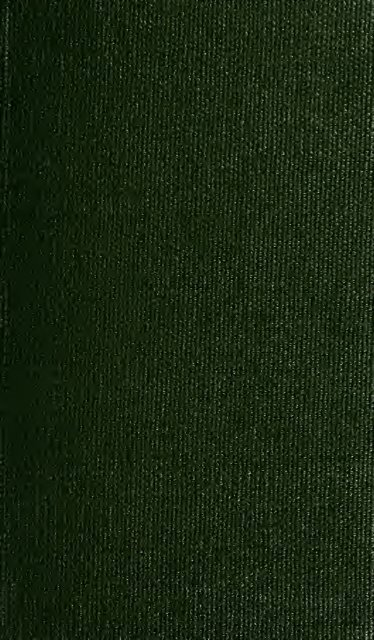The image is a highly zoomed-in close-up of a dark hunter green fabric, featuring a textured surface. It shows a subtle gradient, transitioning from a slightly lighter shade on the right to a darker tone on the left, possibly due to lighting or wear in the material. The fabric appears to be flat and wrinkle-free, set against a white background with no other objects present. Throughout the fabric, small white dots can be observed, which might indicate areas where the color has faded or threads have worn thin. Despite the material's rough texture, it’s difficult to identify the exact type of fabric, but it could be something akin to a rug or carpet. The image's focus on a single piece of cloth without visible context or usage hints keeps the material's purpose ambiguous.